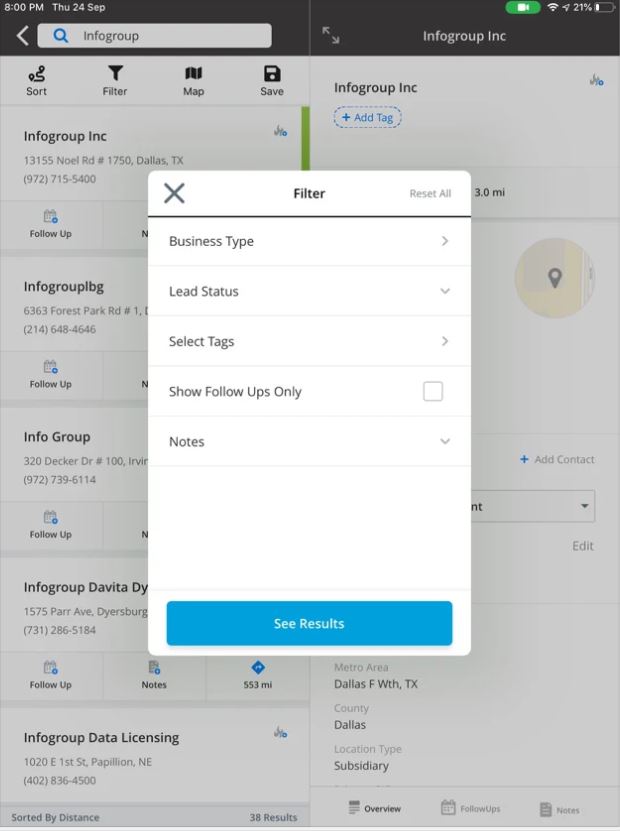This screenshot captures a web search session on a mobile device, where the interface indicates current activity and status details. At the top left, essential information such as the time (8 PM) and the date (Thursday, 24th September) is displayed. Adjacent to this, a search bar labeled "Info Group" with a blue magnifying glass icon signifies the search term input.

The bulk of the screen's real estate contains search results for "Info Group," with entries listed vertically on the left-hand side: "Info Group Inc," "Info Group IBG," "Info Group," "Info Group DaVita," and "Info Group Data Licensing." An ongoing action prompts a visible overlay—a bright white pop-up against a darkened background, suggesting a modal interaction, likely triggered by the user for filtering purposes.

This action places a lighter-colored filter options window in the forefront. The user has interacted with the "filter" button from a toolbar at the top of the search results list, featuring options for "Sort," "Filter," "Map," and "Save." 

On the top right of the screen, a green oval icon with a white camera suggests that the session is being recorded, potentially for documentation like insurance purposes. Additional interface elements such as the battery indicator showing 20% charge provide context to the user's environment during this interaction. This detailed depiction captures both the technical and navigational aspects of the user's browsing experience on a mobile device.